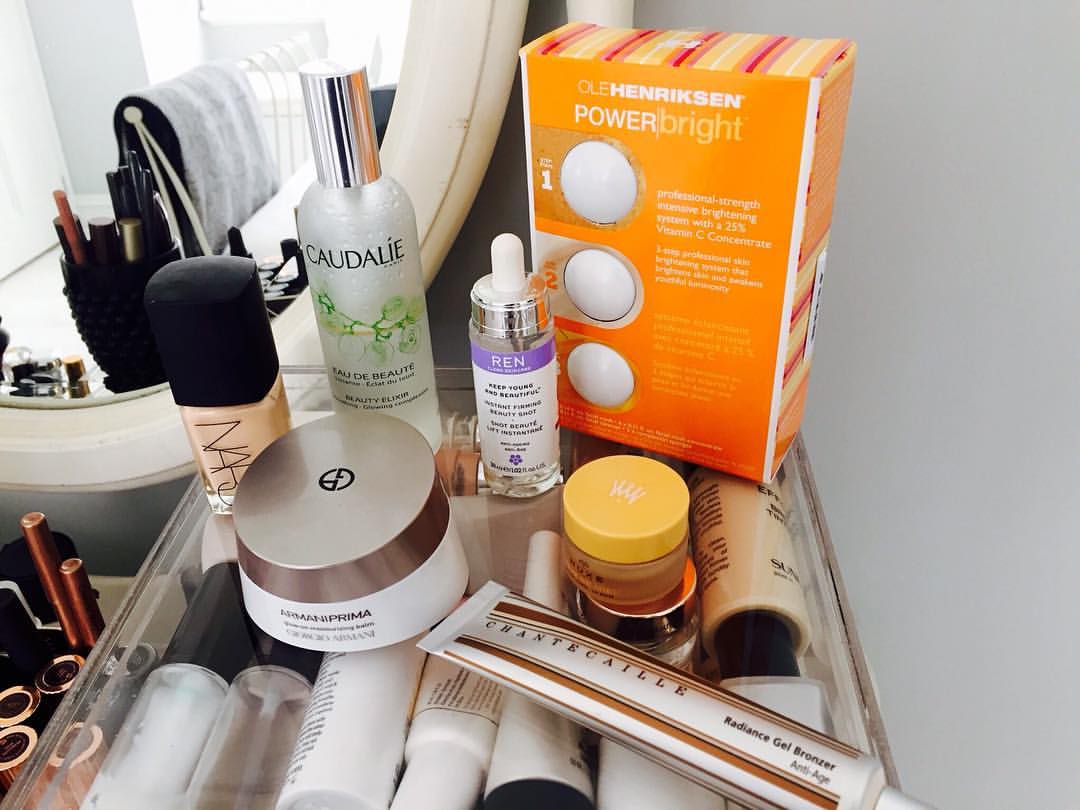A well-organized countertop displays an assortment of beauty supplies, showcasing a comprehensive collection of makeup and skincare products. Prominently featured are several tubes and bottles, containing an array of lotions, facial toners, and cleansers—essential items for any beauty routine. Although many of the labels are not clearly visible, it's evident that these products are typically found in a beauty supply store. Among the items, a large, eye-catching orange box labeled "Ole Henriksen Power Bright" stands out, likely indicating a skincare treatment. Also present is a round, colorful bath bomb, suggesting indulgence in luxurious self-care. Other items on the shelf include mascaras, bronzers, and various other beauty essentials that cater to diverse cosmetic and skincare needs, creating a comprehensive display of personal beauty requisites.